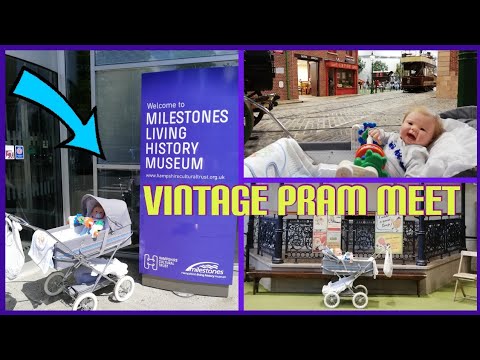The poster, dominated by a black background with substantial letterboxing on the top and bottom, is divided into three distinct sections by thin purple lines. The entire poster is framed by this same purple outline. The yellow text "Vintage Pram Meat" spans the middle of the overall layout. 

On the left, there is a purple billboard sign with white text that reads "Milestones Living History Museum" accompanied by an image of an old-fashioned baby carriage. This carriage is gray with an awning, white wheels, and a handle for pushing. An arrow points down at the baby inside the carriage.

To the right, the poster is split into two rectangles. The upper right section shows a baby lying in a stroller with a gray cover, facing the camera and appearing to cry. The lower right section features the same gray stroller from a different angle, this time in front of an iron fence, with the baby turned towards the three o'clock position. The baby in these images has a white blanket around them and blonde hair. 

The overall layout distinctly presents a vintage theme, connecting the elements through a uniform purple hue and consistent stroller imagery.